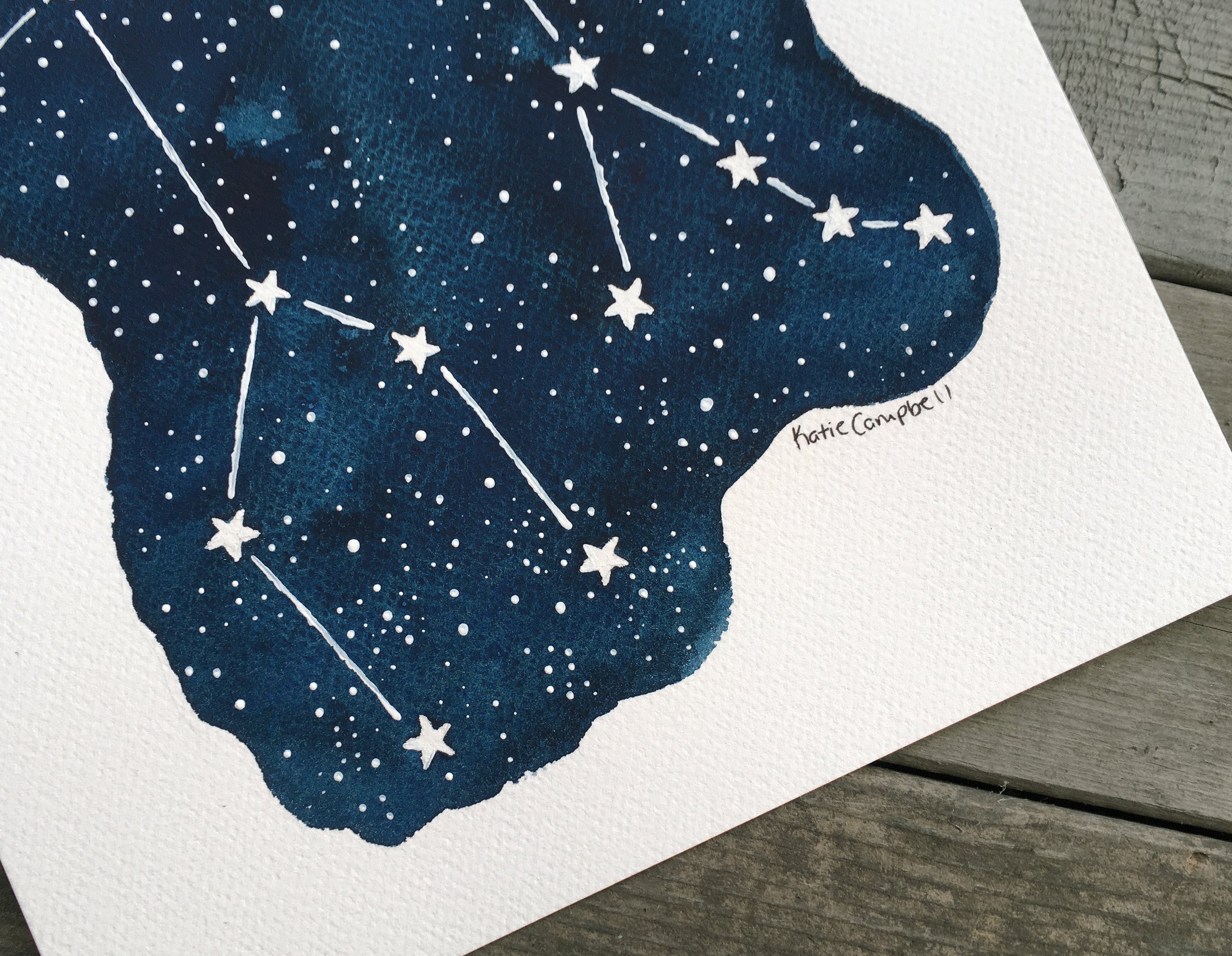This image depicts a beautiful watercolor painting by Katie Campbell, signed in small black letters at the bottom. The painting, done on textured cardboard paper, features a deep blue sky with varying shades from dark to light. Adorning the sky are numerous white stars, some represented as simple dots and others with five-point shapes. Among these stars, two constellations are illustrated with connecting lines, each constellation composed of five stars forming distinct patterns. The painting exudes a cosmic theme, capturing the essence of space with its minimalist but detailed portrayal. The background of the image shows wooden planks, suggesting the painting is photographed on an outdoor table or deck, with the artwork front and center on a white canvas.